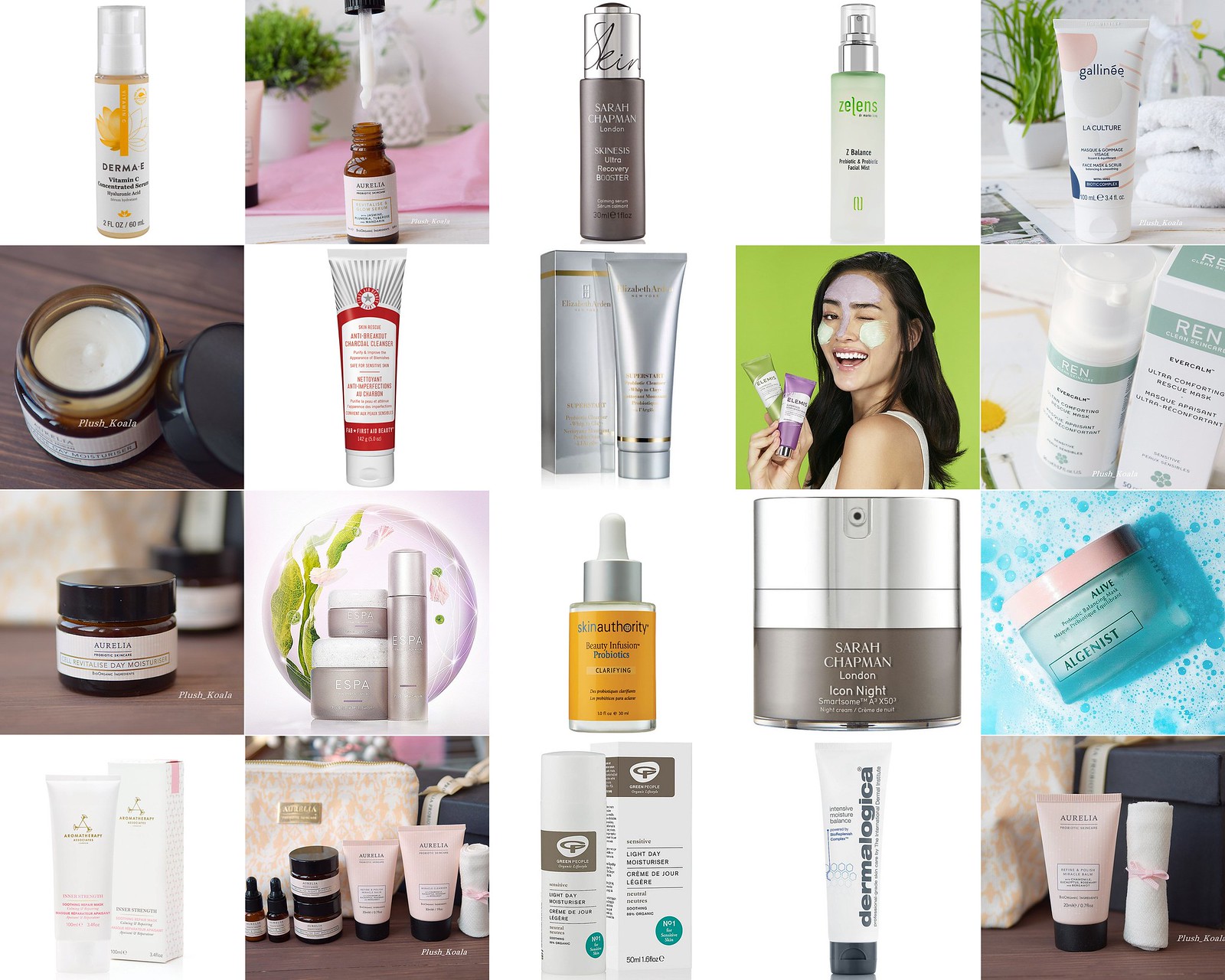This image features an organized collage of 20 distinct makeup and skincare products, arranged in a grid resembling a Pinterest board. Each square showcases a different item, creating a visually appealing and comprehensive overview. 

Starting from the top left, the first item is a white foamed container accented with a yellow stripe. To its right is a brown bottle set against a pink background. Next, there is a sleek gray bottle with a silver cap, followed by a green bottle also adorned with a silver cap. Concluding the first row is a tube placed on a countertop.

In the second row, beginning from the left, there’s an open cream jar with its lid off. Next to it is a vibrant red tube, followed by a silver tube decorated with white and red accents. Adjacent to this is another plain silver tube.

The fourth image in this row diverges slightly, featuring a smiling woman with face cream applied and two dots on her cheeks, adding a human touch to the collection. This is followed by an image with a green background showcasing a couple of tubes, one purple and one green. 

The final slot is occupied by a white container. Additional various tubes and bottles, differing in shapes and sizes, fill other squares. The entire grid is evenly spaced, providing a structured and aesthetically pleasing layout.